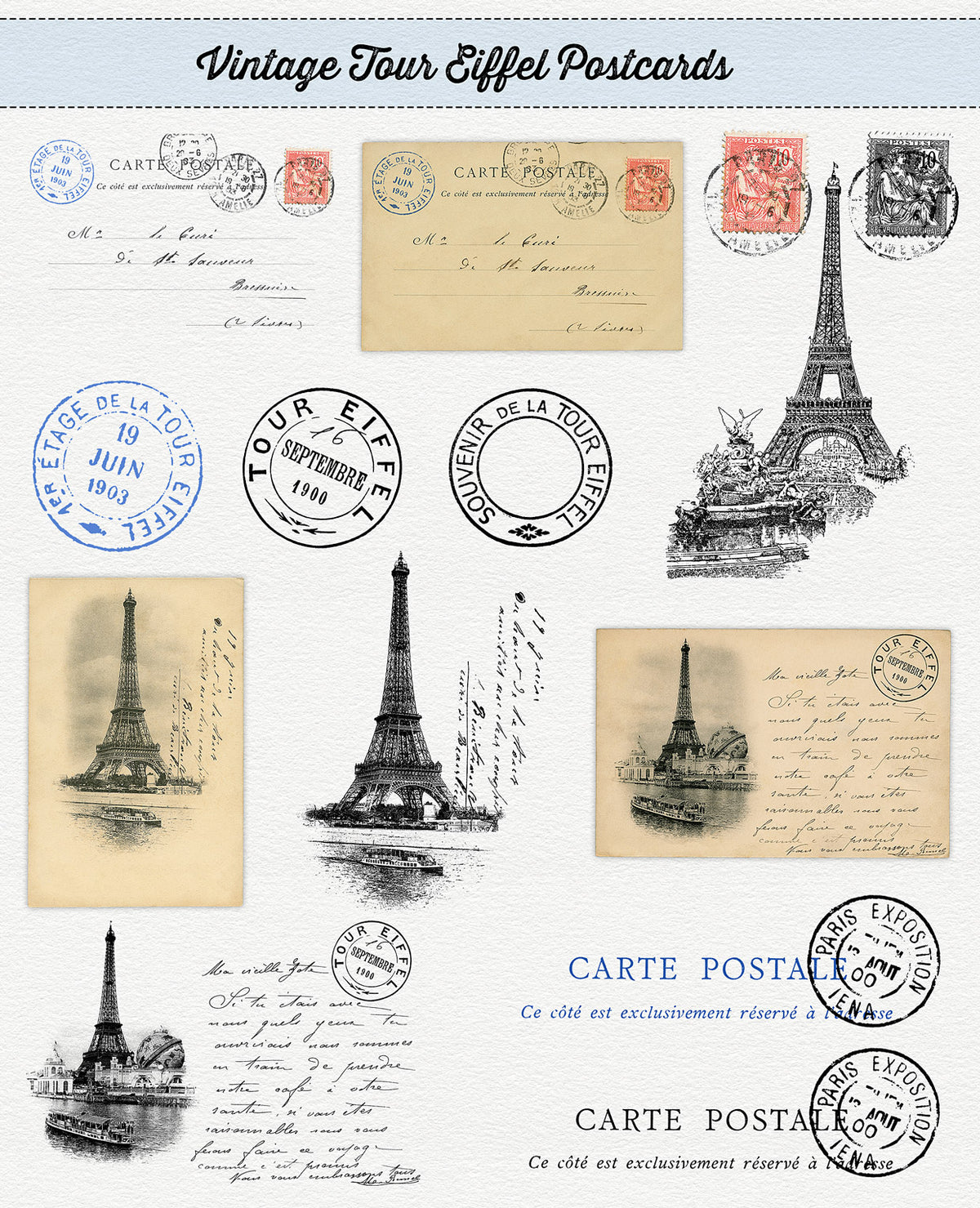This image captures a fascinating collection of vintage Eiffel Tower-themed postcards displayed on a white background. Across the top, bold black letters announce "Vintage Tour Eiffel Postcards." These postcards, bearing an array of ornate postage marks, radiate an antique charm. The meticulously arranged assortment includes postcards in various shades — from discolored tan-brown hues to pristine white — each emblazoned with imagery of the Eiffel Tower. Among them, a postcard stands out with elegant cursive handwriting, resembling a letter. Scattered throughout are diverse postage stamps: some round, others square, with cancellation marks in black and blue ink. Red and black stamps accentuate the aged aesthetic. Noteworthy details include postal marks reading "Cartier Post" and "Cartier Postel," alongside postcards dated as early as 1900 and 1903, all underscoring the nostalgic essence of this timeless collection.